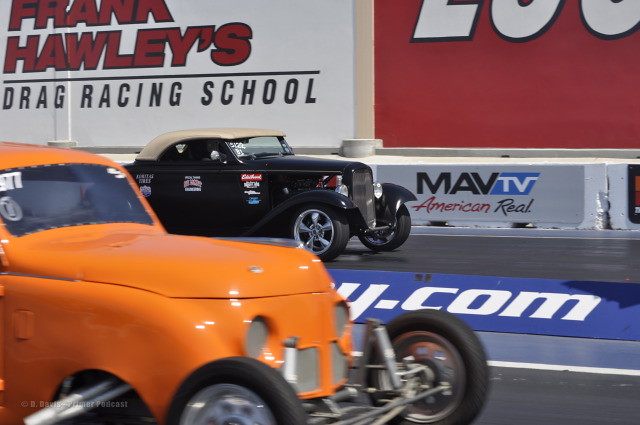The image captures an exciting moment at a classic car drag race on a racetrack, clearly demarcated by several signs in the background. To the left, there is a sign for "Frank Howley's Drag Racing School" in red and black letters, while another large red sign with unreadable white letters can be seen to the right. Central to the scene is a prominent "MAV TV American Real" sign. The car closest to the camera is a vibrant orange T-Bird, equipped with narrow racing tires and extended axles projecting from the front. This car exudes a vintage flair consistent with the hot rod genre. Opposite it and slightly behind, there is a black convertible styled with an old-school grill and a white top. This vehicle, also covered in sponsor logos along the passenger door, shares the same classic design as the orange T-Bird. Though the specifics of the sponsors’ messages are indistinguishable, the scene is lively and evocative of a bygone era of drag racing.